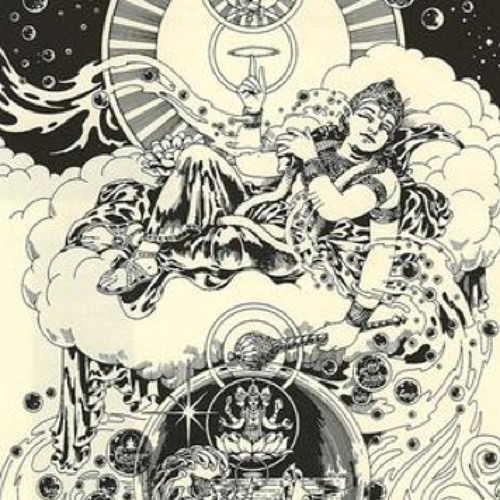This is a detailed black and white illustration that appears to depict a Hindu deity, characterized by multiple arms. The image is vertically rectangular with no specific border or background. The upper left and right corners are heavily shaded in black with bubble-like patterns. At the center, a deity is depicted reclining on a cloud, eyes closed, seemingly in a state of rest. One arm is pointing upward towards a circle, possibly a halo, while another arm holds a scepter that also features a halo. Below this, the same deity is portrayed in a face-front position, with six arms arranged in meditative poses, seated in a lotus flower. The rest of the image is filled with intricate swirls and abstract designs, contributing to its overall artistic and interpretive nature, possibly as an homage to Hindu iconography.